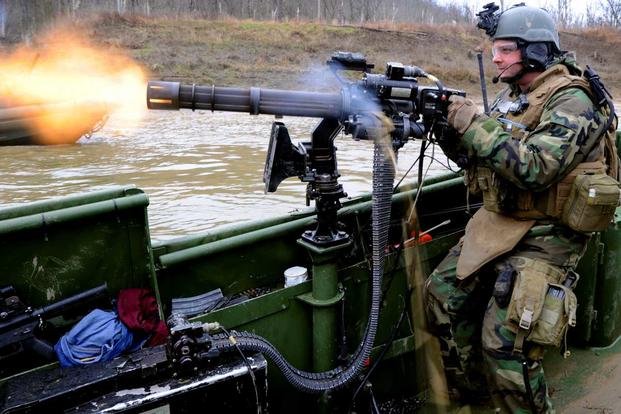In this dynamic photograph, a soldier is seen actively using a mounted machine gun on a small, green-painted boat amidst an outdoor setting. The soldier, positioned on the right side of the image, is seated and gripping the handles of the machine gun, which is being fed by a long chain of bullets. Clad in an extensive array of gear, including a bomb protection jacket, helmet with microphone, gloves, and several bags attached to his sides and hips, he embodies a fully-equipped and alert combatant. Additionally, he is wearing goggles and headphones, highlighting the need for secure communication and protection.

The gun is in action, emitting orange-red muzzle flashes and smoke where the ammunition feeds into the machine. The surrounding environment features a water body that appears muddy and brown, with relatively calm waters and a forested riverbank in the background. The riverbank is steep and mostly bare, indicating a woody area transitioning into late autumn or winter. The trees are notably devoid of leaves, and the grass on the hill is a mix of brown and sparse green. The scene captures a tense moment of military activity set against the muted, natural backdrop.